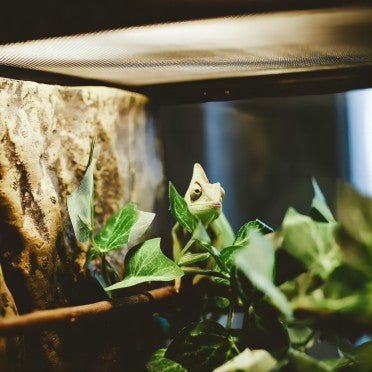This detailed close-up image captures a Jackson chameleon residing in its terrarium. The green chameleon, with its distinct, pointed head and black eyes, is positioned on a branch adorned with artificial leaves, slightly obstructing its body. The chameleon's head is oriented upward and slightly to the right, away from the camera's view. Overhead, a dimly lit terrarium light illuminates the scene. To the left, a faux stone wall prevents the chameleon from climbing out. The background reveals a hint of the surrounding room, blurred to emphasize the chameleon. The terrarium's transparent walls contribute to the clarity of the image, spotlighting the chameleon as the central focus.